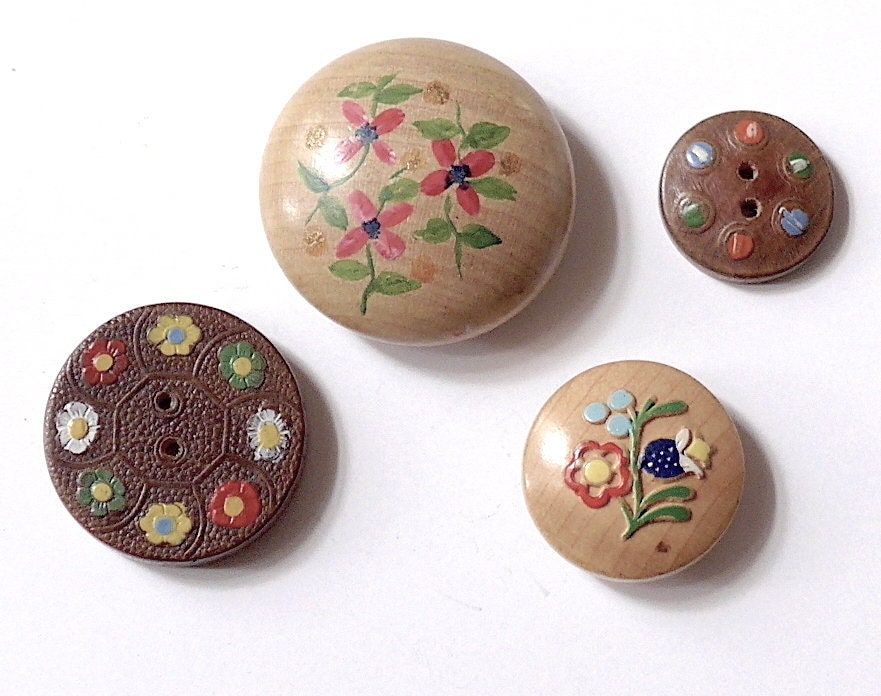This is an indoor color photograph depicting four intricately hand-painted circular wooden objects, likely buttons or knobs. The bottom left object is a dark brown circle with two small central holes, surrounded by alternating colorful flowers: yellow with a blue center, green with a yellow center, white with a yellow center, and red with a yellow center. The top middle object is a larger wooden knob painted with three flowers having green stems, pink leaves, and black interiors. The top right object is another dark brown circle with two central holes and painted dots around the perimeter in green, red, and blue. The bottom right features a smaller wooden circle adorned with a painted green stem, a red flower with a yellow center, two light blue dots, and a blue flower with a yellow center. Each object contributes to a vibrant and detailed composition, emphasizing the intricate craftsmanship and colorful design.